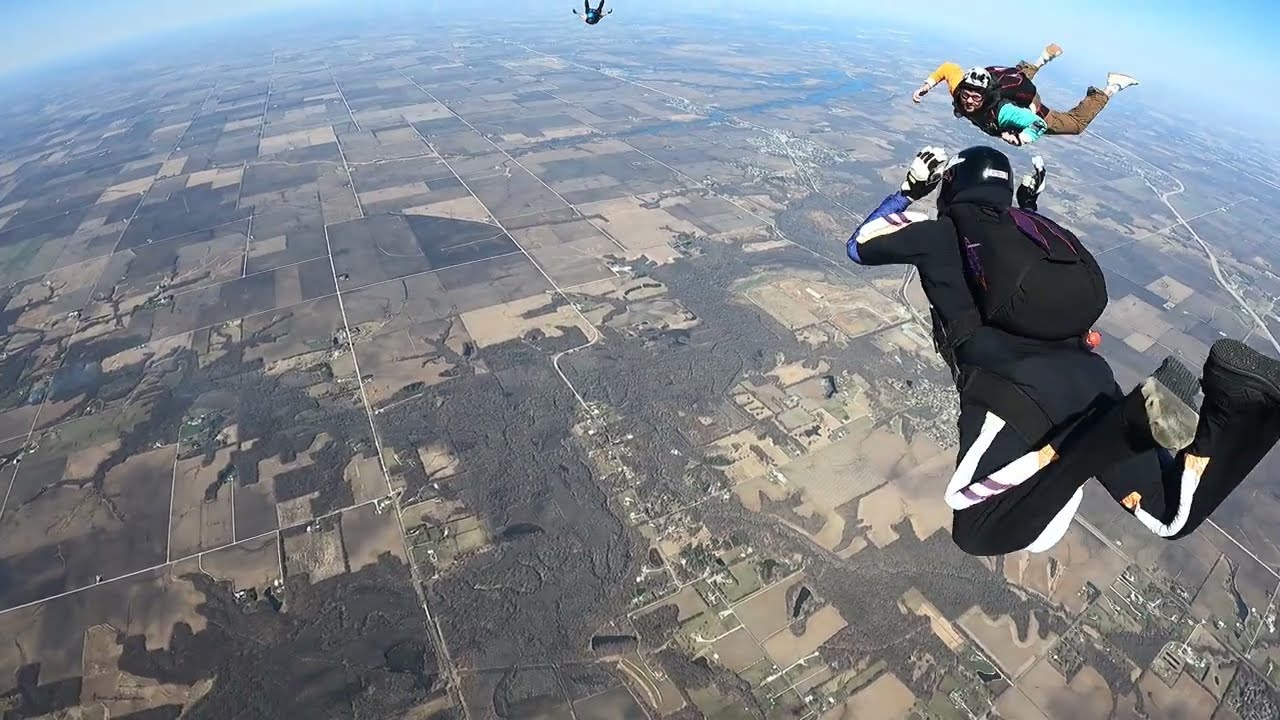A breathtaking full-color aerial photograph capturing the thrilling moment of three skydivers plummeting through the sky. The vantage point is high above the earth, possibly around 10,000 feet, offering an expansive view of the landscape below, which includes roads, fields, scattered trees, and occasional buildings. The curvature of the earth is visible, suggesting the immense height at which the photo was taken — possibly by a fourth skydiver who captured this incredible scene.

In the foreground, a skydiver dressed in a sleek, black professional jumpsuit with white accents and white gloves is prominently visible, their parachute backpack strapped securely. To the right of this skydiver, another diver wears a more casual skydiving ensemble consisting of brown pants, a turquoise and yellow shirt, and a helmet with goggles, creating a striking contrast against the more uniform look of the other divers. The third skydiver, seen further in the distance, appears to be clad in a blue helmet and dark jumpsuit, though the exact details are less discernible due to their position.

The photograph, taken during the daylight with the sun high in the sky, possibly early evening, beautifully captures the essence of skydiving and the boundless horizon stretching out below.